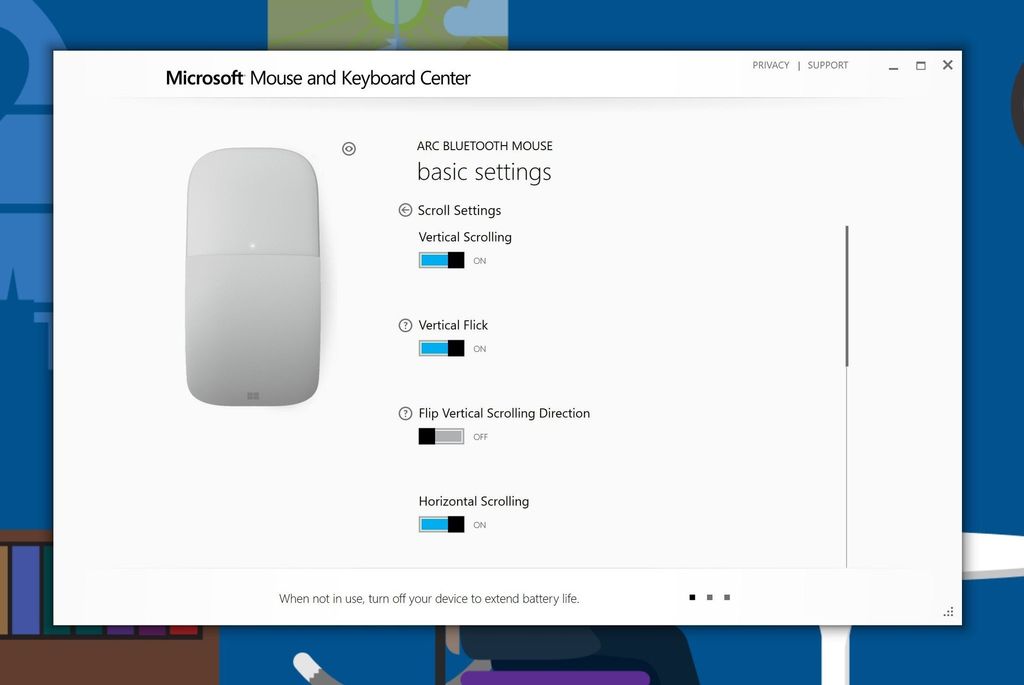The image displays a pop-up that takes up most of the background. In the upper right-hand corner of the pop-up, the background is light in color while the text "Privacy" appears in gray. A vertical line divides the text, leading to a button that resembles an underscore, likely used to minimize the window. There's also a box for expanding the window and an "X" for closing it.

On the left side within the pop-up, "Microsoft" is prominently displayed in bold black text, followed by "Mouse and Keyboard Center" in regular black font. Below this, a gray mouse graphic is partially depicted, showing about half of its shape.

Beneath the graphic, various mouse settings are listed:
- "Arc Bluetooth Mouse" followed by sections on "Basic Settings" and "Scroll Settings."
- "Vertical Scrolling" is noted to be "on," indicated by a blue line.
- "Vertical Flick" is also "on," marked similarly with a blue line.
- "Vertical Flip" and "Vertical Scrolling Direction" are mentioned but with a gray line.
- "Hover" is toggled on, detailed in black text with an accompanying blue line.

A thin gray line extends across the pop-up, underneath which it advises in gray text, "When not in use, turn off the device to extend battery life."

At the bottom, three squares are displayed: one black, one dark gray, and a slightly lighter dark gray. 

The background behind the pop-up is a blend of different colors, including purple, blue, brown, red, green, and white, though details of the background are obscured by the pop-up itself.